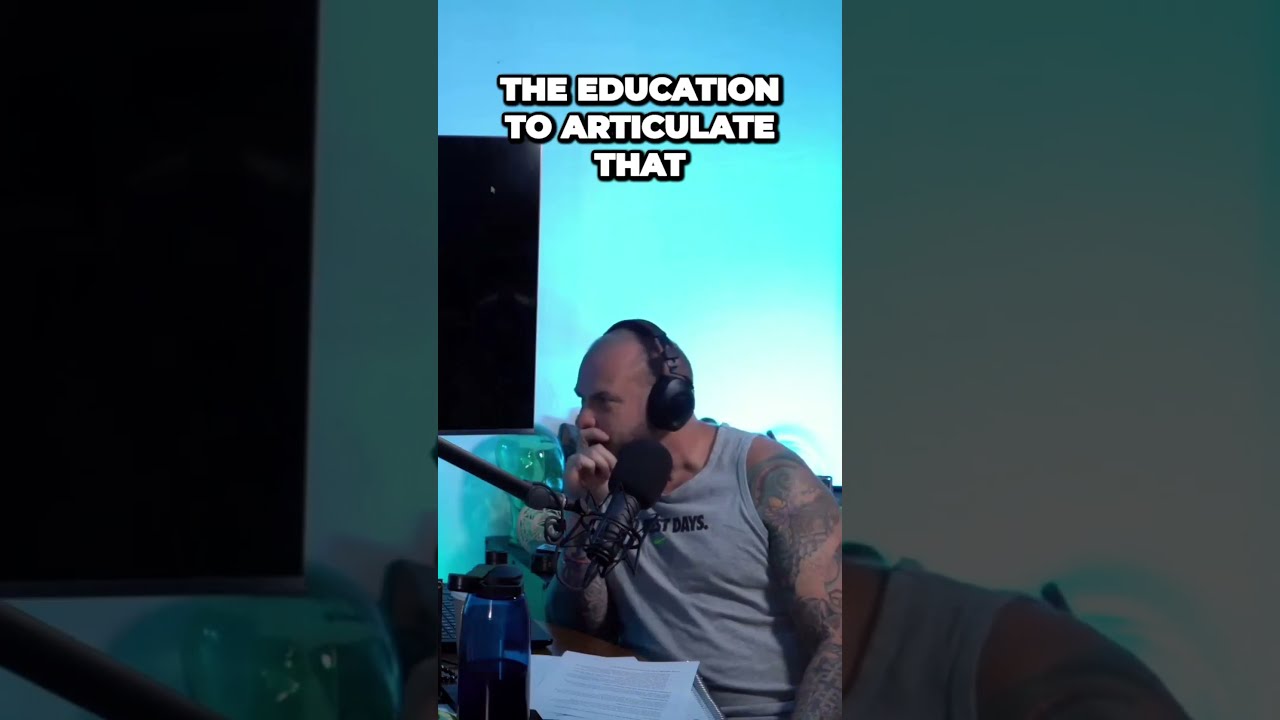The image centers around a bald, middle-aged Caucasian man with a well-built, muscular frame, adorned with a sleeve of tattoos on his left arm. He is wearing a gray Nike tank top, featuring some black lettering with the visible words "seven days," and a light green check mark. The man, sporting over-the-ear black headphones, sits at a desk in front of a large microphone attached to a boom arm, a monitor, a stack of white papers, and a clear blue plastic water bottle with a black cap. His chin rests on his right hand, giving him a contemplative look.

The background is a creatively enlarged, dimmed, and faded portion of the same photograph, giving the entire frame a cohesive, layered appearance. The right and left thirds of the background display an extended image of the man's shoulder and a TV screen, respectively, both merged smoothly into the darker overall tone. The upper part of the frame reads "the education to articulate that" in white font with black shadowing, suggesting this might be a screenshot taken from a Reel or TikTok video designed for mobile viewing, given the aspect ratio and layout. The atmospheric backdrop in a muted blue hue, paired with the thoughtful pose of the man, adds a reflective ambiance to the scene.